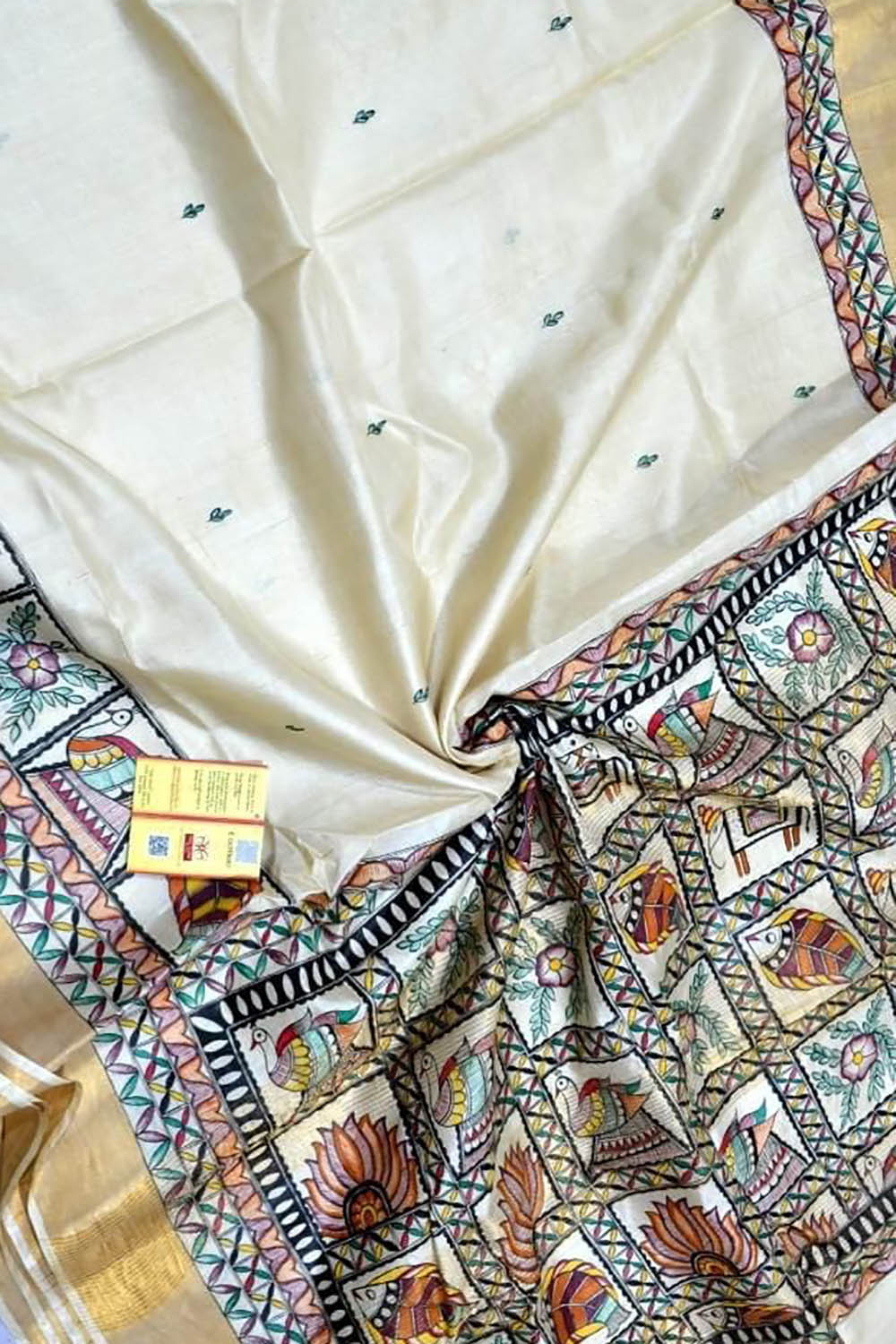This image features a scarf that is laid out on the floor, with the center portion slightly gathered to create a circular, rippling effect. The fabric is thin and delicate, bearing a combination of both understated and vibrant details. The upper section of the scarf is primarily a light tan or cream color, adorned with small, scattered leaf designs. In stark contrast, the bottom section of the scarf is richly decorated with colorful, intricate patterns that seem inspired by Asian or Indian art. 

This vivid border includes recurring motifs positioned in squares: a multicolored bird with rainbow-like feathers, a variety of brightly scaled fish in shades of orange, red, and yellow, and a series of flowers in hues of purple, orange, and red. Additionally, there are swirling designs in blue, purple, and yellow, framed by gold accents. Each motif is distinct yet harmoniously contributes to the eye-catching, artistic flourish of the scarf’s design.